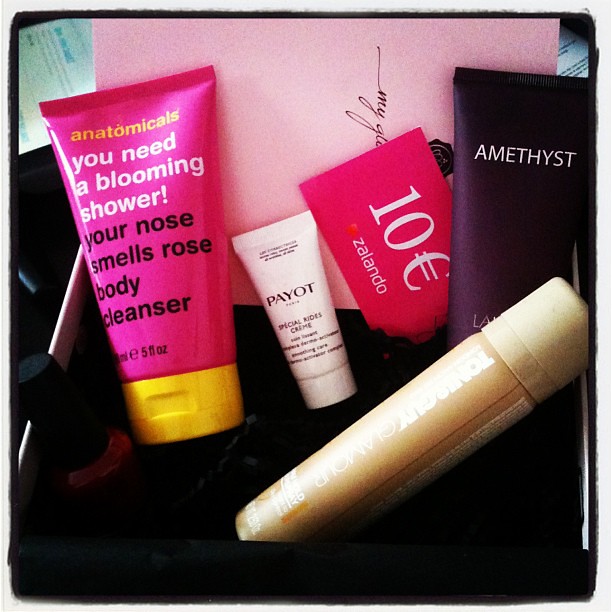This is a full-color photograph showcasing a well-built gift box placed against a light gray background. The box features a gray and black marbled base, with the main box itself being black with a raised edge. Inside, it holds several beauty supplies. Prominently, there is a dark pink card with black cursive writing, only the word "my" is legible. Among the items, there is a notable body cleanser from Anatomicals, labeled "You need a blooming shower, your nose smells rose," featuring a pink tube with a yellow cap and white and black text. Adjacent to it, there is a white tube of special cream from PAYOT, although the smaller text is difficult to discern. A black rectangular box of Amethyst skincare sits nearby, along with a tan tube of what appears to be lipstick in the lower right corner. Additionally, there is a partially visible coupon for 10 euros from Zalando, identifiable by the "1-0" in white numbers on a dark pink background, tucked into the lower left corner of the box.